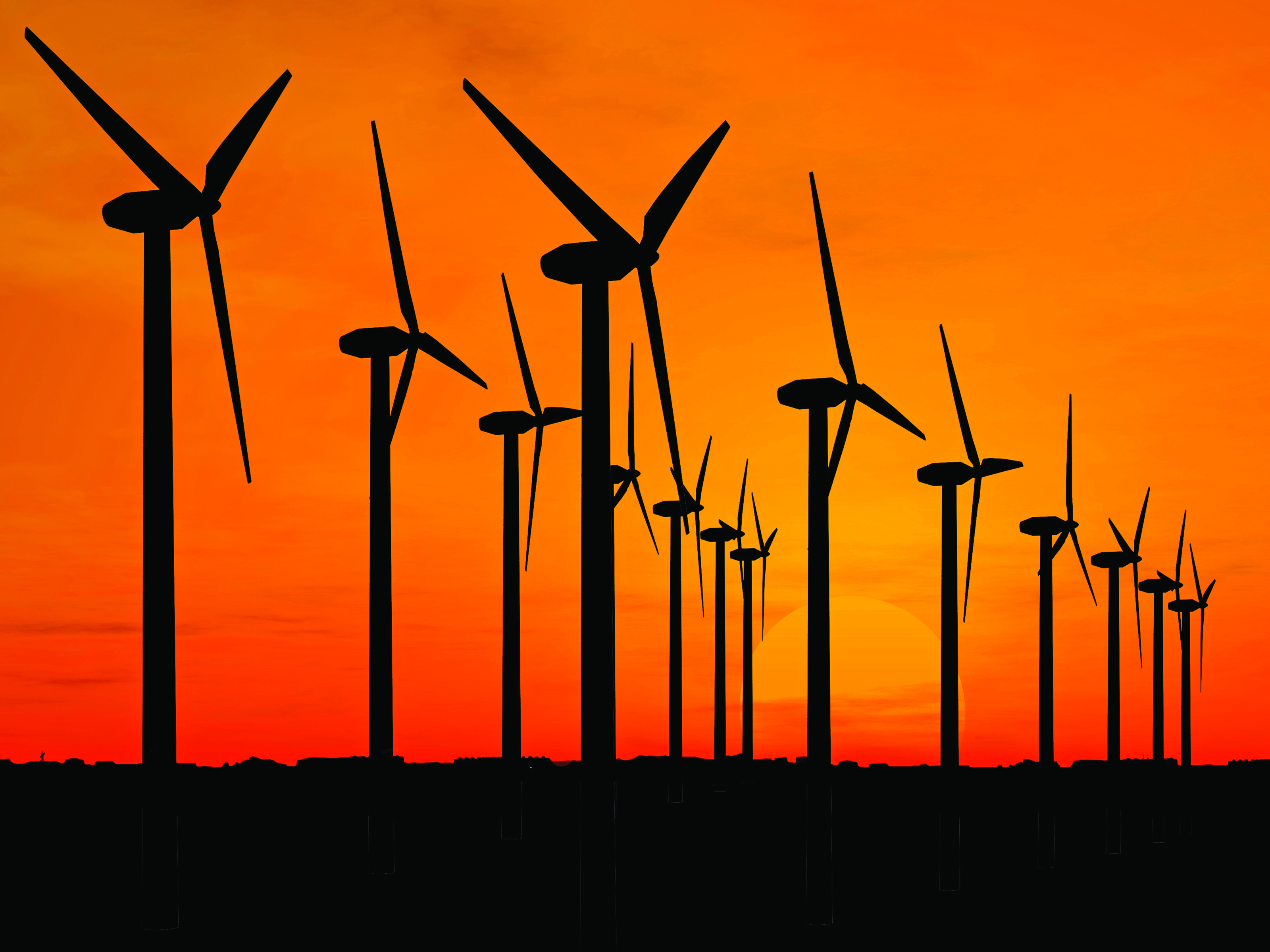In this photograph taken at sunset, a row of about 10 windmills stands solemnly against a sky ablaze in fiery shades of yellow, orange, and red. The ground and the windmills appear as dark silhouettes, creating a stark contrast with the vibrant hues of the evening sky. The sun, positioned just above the horizon, casts a yellow glow, partially obscured by some thin strips of clouds. Each windmill, aligned in two organized rows, features three long blades resembling slender, straight-topped triangles, reminiscent of jet airplane wings. The bottom portion of the image is predominantly black, emphasizing the grand stature of the windmills as they rise from the darkened ground into the colorful twilight.